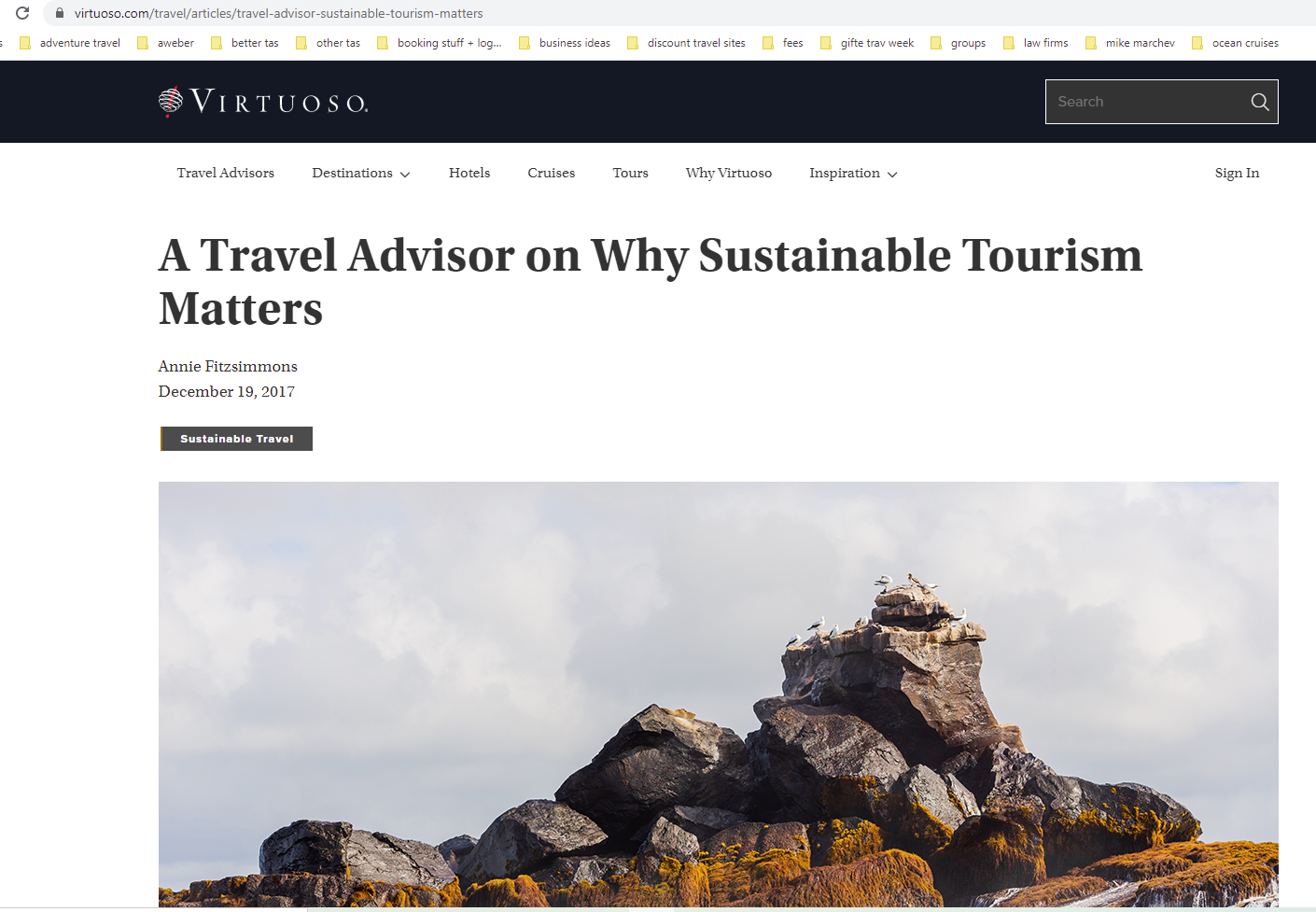A detailed caption for the described image:

"Screenshot from the Virtuoso website featuring an article titled 'A Travel Advisor on Why Sustainable Tourism Matters' by Annie Fitzsimmons, dated December 19, 2017. The webpage includes navigational buttons for travel adventures, destinations, hotels, cruises, and tours, along with an option to learn 'Why Virtuoso?', a sign-in button, and a search bar. The accompanying outdoor photograph showcases a dramatic cloud-covered sky highlighting a series of large rocks adorned with patches of orange-colored moss. Atop the highest rock perch around ten birds, predominantly white with some featuring gray markings, creating a striking scene above the rugged landscape."